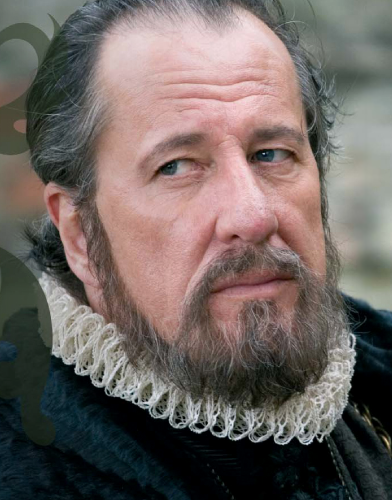In this image, an older man is prominently featured at the center, capturing most of the frame with his face and the very top of his chest. The background is blurred, hinting at an outdoor setting, likely in daylight. The man is depicted with a receding hairline, dark hair interspersed with gray, slicked back into a rounded shape. He has blue eyes that are looking seriously off to his right, even as his body faces slightly left. His long, thin face is adorned with a mustache and a somewhat lengthy beard. He wears a historical outfit resembling attire from the Middle Ages or Renaissance, characterized by a white, fluffy ruffle collar around his neck. The color palette of his clothing includes black, blue, and very pale beige, adding to the period costume's layered and textured appearance. The background on the right side appears lighter, while the left side is darker, enhancing the focus on the man's expressive features and elaborate costume.